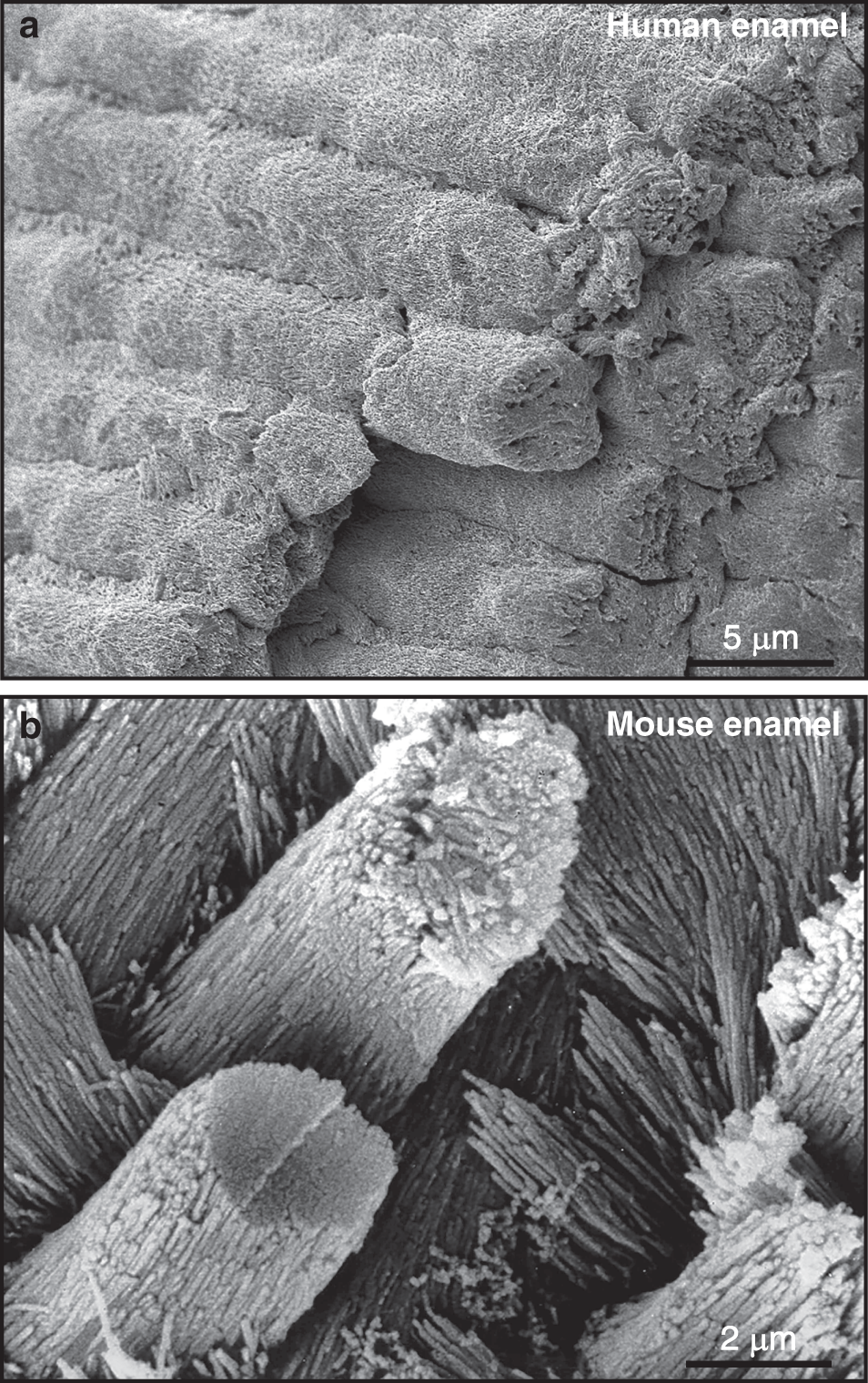The image is a rectangular graphic measuring about 6 inches high and 3 inches wide, featuring two black-and-white photographs stacked vertically. Each photo is bordered by a thin black line and separated by a white horizontal divider. 

The top photograph depicts human enamel and is labeled with a lowercase letter 'a' in the upper left corner. The upper right corner displays the text "human enamel" in white print. The lower right corner features the measurement label "5μm" in white print with a black underline. This image shows a microscopic view of human enamel, characterized by light gray, tubular structures resembling long rolls of hay, with sponge-like ends.

The bottom photograph portrays mouse enamel and is labeled with a lowercase letter 'b' in the upper left corner. The upper right corner reads "mouse enamel" in white print, and the lower right corner displays the measurement "2μm" in white print with a black underline. This image reveals a microscopic view of mouse enamel, displaying thin, cylindrical bands or clumps that resemble brittle wood or stalagmites, with varying shades of gray suggesting a less uniform, more spiky formation compared to the human enamel above.